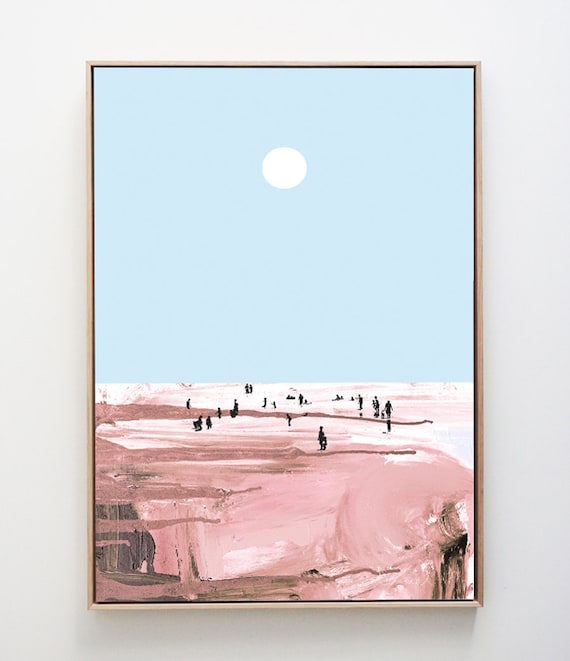This detailed image depicts an oil painting, or a reproduction thereof, hanging on a white wall surrounded by a thin light-colored frame, possibly metal or wood. The painting is dominated by a vast, clear blue sky that takes up more than half of the canvas. Central in the upper part of the sky is a luminous white celestial body, which could be interpreted as either a sun or moon. 

The lower portion of the painting represents land, painted in various shades of pink and light brown, with streaks of darker pink and brown running horizontally. This terrain appears to be either a desert or the surface of a canyon, characterized by a clay-like texture. Interspersed across this pink-hued ground are numerous tiny black figures. These figures, which could be people or native inhabitants, appear to be walking or milling about, with some in pairs and others alone. A couple of these figures even seem to have small animals with them. The overall scene evokes a sense of solitude and sparse movement, set against a strikingly simplistic yet evocative backdrop.